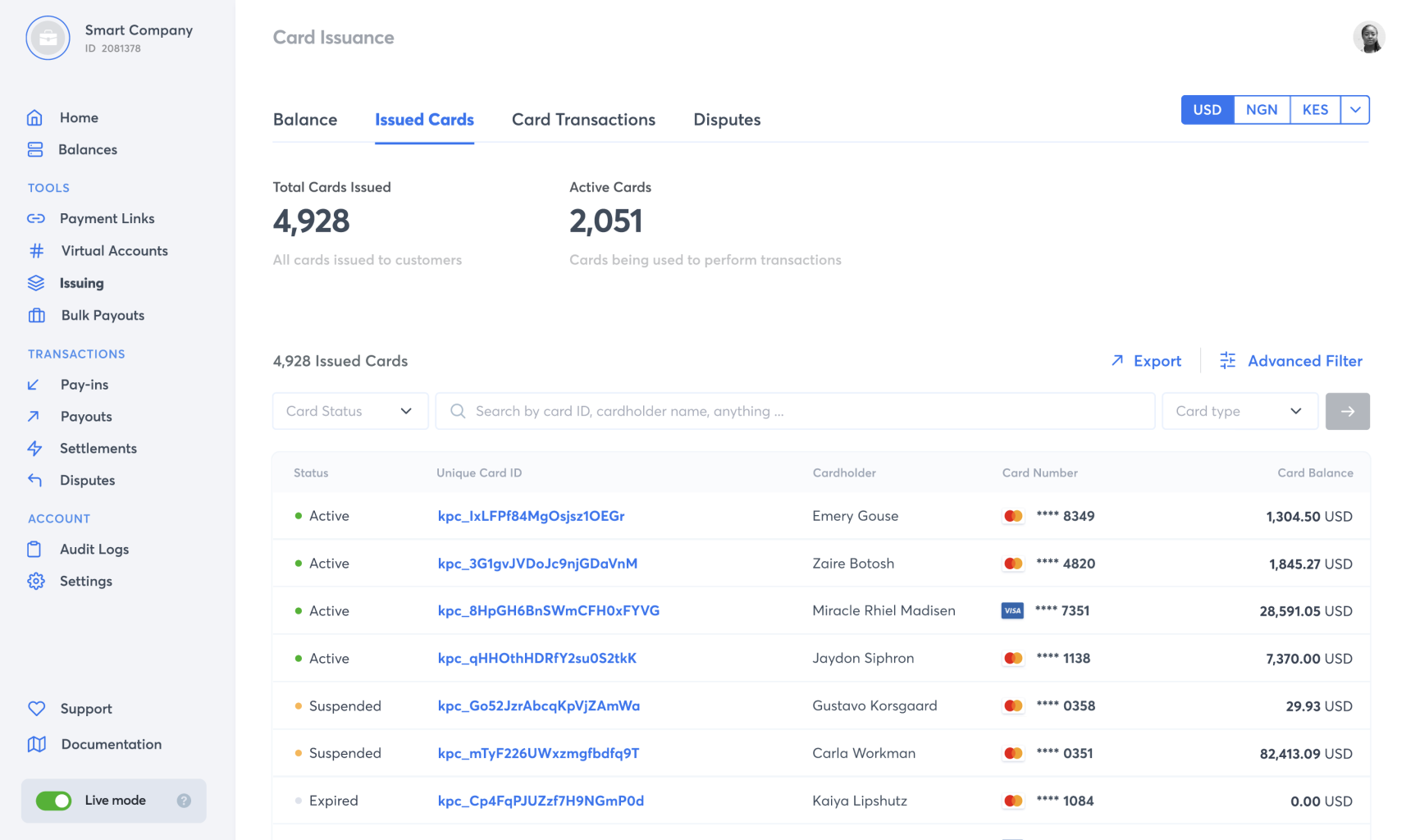Sure, here is a more detailed and cleaned-up caption:

---

The interface of Smart Company's dashboard (ID: 2081378) is displayed in this image. On the left, there is a vertical navigation bar with a gray background and black text. The options listed in the navigation bar are: Home, Balance, Tools, Payment Links, Virtual Accounts, Issuing, Bulk Payouts, Transactions, Pay In, Pay Out, Settlements, Disputes, Account, Audit Log, Settings, Support, Documents, and Live Mode.

On the right side of the dashboard, the focus is on Card Issuance and Balance management. There are several tabs available, including Balance, Issued Cards, Card Transactions, and Disputes. The tab for "Issued Cards" is currently selected, showing detailed statistics and information about the cards issued.

At the top of this section, it states "Total Cards Issued: 4,928," and further breaks it down with "All Cards Issued to Customers" and "Active Cards: 2,051." These cards are used in platform transactions.

Below the summary, there is a search bar allowing users to search by Card ID, Card Holder Name, or other criteria. The status of the cards is indicated with a green dot for active cards. Each card entry includes details such as Unique Card ID, Card Holder Name, Card Number, and Card Balance. 

The displayed list shows the first seven entries:
1. An active card with cardholder Emery Grouse, a MasterCard ending in 8349.
2. Another active card with cardholder Zary Grosh, a MasterCard ending in 4820.

---